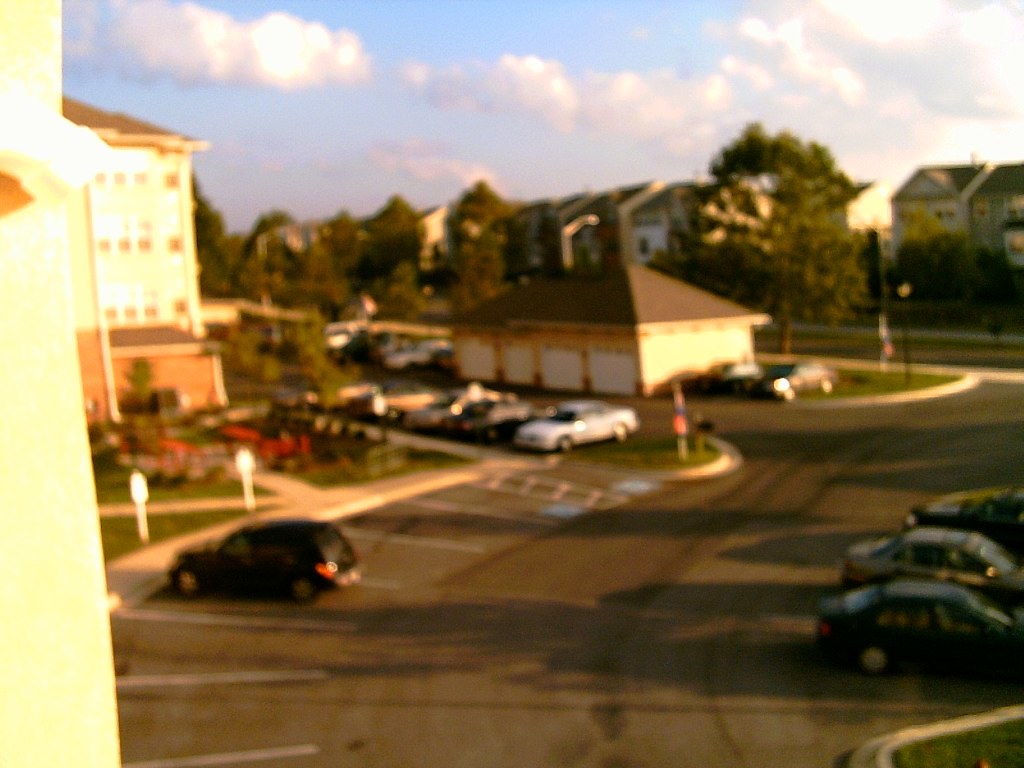This photo, taken from a second or third story window or balcony, captures an aerial view of a condominium complex. The image is somewhat blurry, but the details are discernible. The parking lot below has white painted lines marking the spaces, with some cars parked on both sides. Notably, there's a small black car parked on the left side and a few other cars on the right.

Directly opposite, you see a building with four white garage doors, which appear to belong to one of the condominium units. The scene extends to show a tree-lined street in the distance, beyond which similar-looking condominiums are visible. The sky is blue with a few clouds, suggesting it's a sunny day and likely not winter. Sidewalks crisscross the area, connecting the parking lot to the buildings and forming a Y-shape path towards the road. No text is visible in the photo, making it a pure visual representation of this quiet, residential neighborhood.